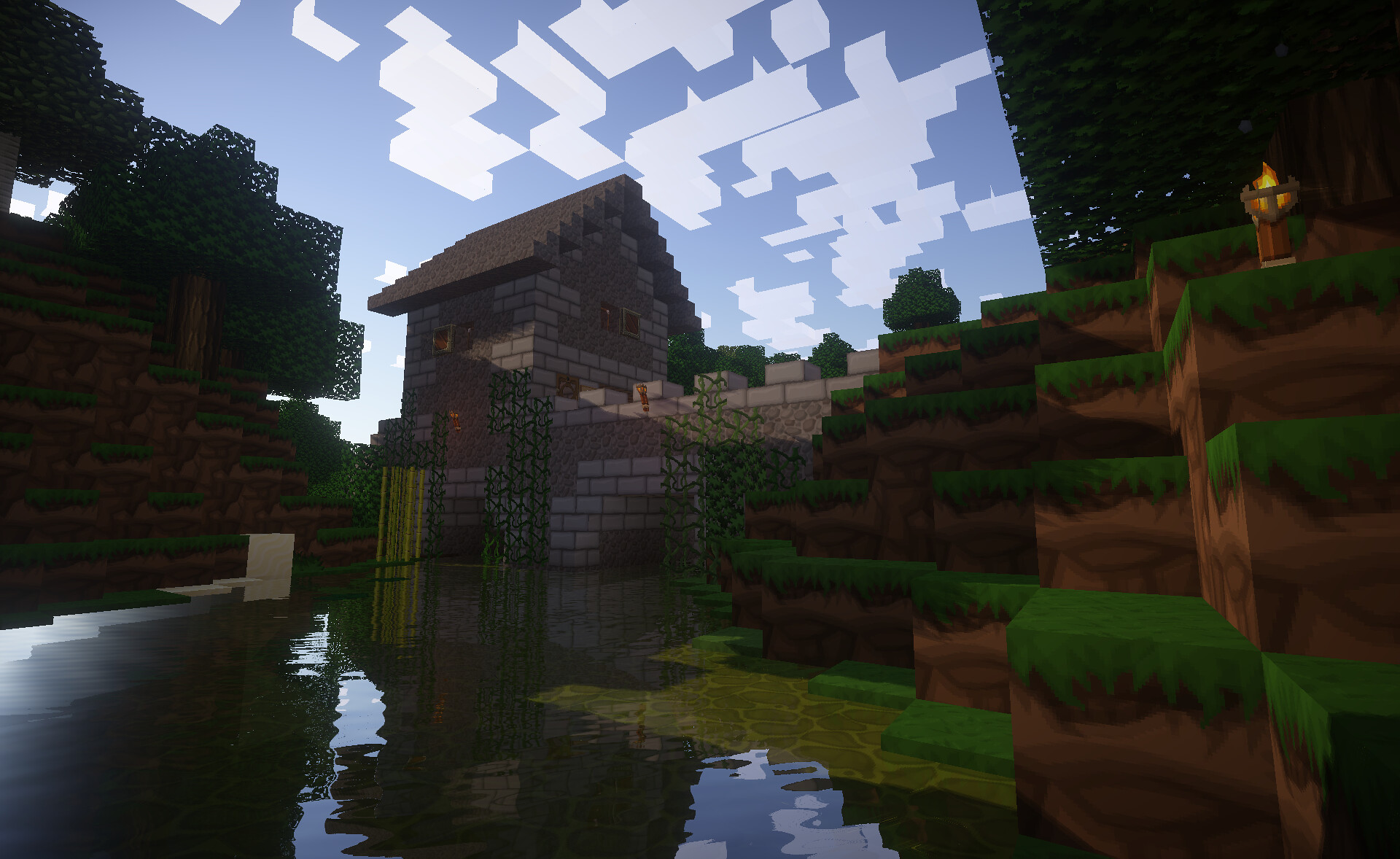This is a highly stylized, color image that appears to be generated by AI, a CAD drawing program, or as part of a video game environment. The scene presents a distinctly blocky aesthetic, reminiscent of voxel art, where objects are crafted from exaggeratedly cubic forms.

In the foreground, a blocky hill emerges on the right side, constructed from layers of green steps and brown earth, culminating in a lantern perched at the top right corner, casting a soft yellow light. The hill overlooks a body of water whose surface reflects light in similarly blocky patterns. 

Dominating the center of the image, a house constructed from brown rectangular blocks sits with a matching blocky roof. To the left, darkened, shadowy trees exhibit the same cuboidal edges, interspersed with block-like leaves.

Above, the sky is a clear blue, dotted with squarish and rectangular white clouds, further emphasizing the uniform blocky theme. The overall composition emanates an unfinished feel, as if part of a digital world still in the process of being built. The level of detail in the blocky design conveys an almost playful yet intricate simplicity, capturing the essence of a digitally created landscape.